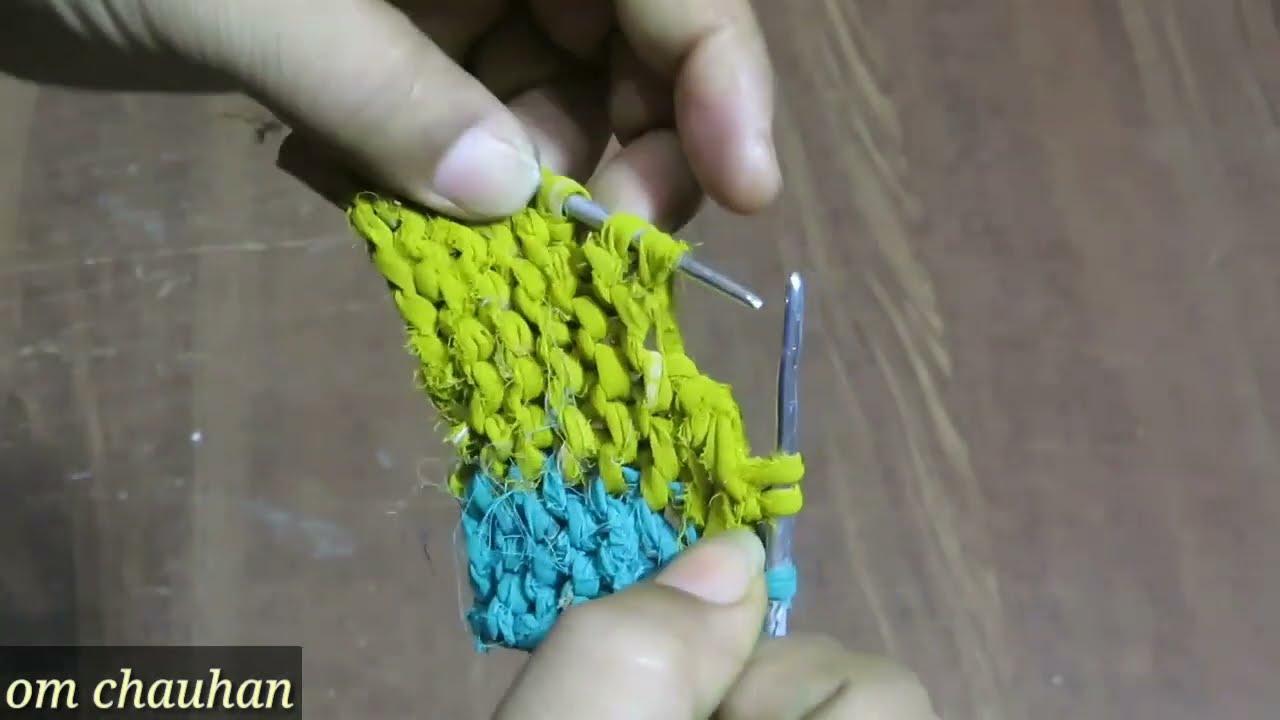In this top-down image, two hands, possibly feminine, are prominently positioned at the center, holding stainless steel knitting needles and working on a partially completed knitted piece. The fabric features a striking contrast, with the top section in a vibrant lime green and the bottom section in a calming teal blue. The background appears to be wood paneling, likely a tabletop or floor, in various shades of brown, but the natural colors are somewhat distorted, probably due to a filter affecting the white balance. In the lower left corner, a black rectangular overlay with white, all-lowercase text reading "om chauhan" (O-M C-H-A-U-H-A-N) is visible, suggesting a connection to a possible DIY or how-to knit channel, possibly on YouTube. The hands display precision, with the thumb and forefinger of the right hand and the thumb, forefinger, ring finger, and middle finger of the left hand clearly visible, meticulously crafting what may be a rug or similar item.